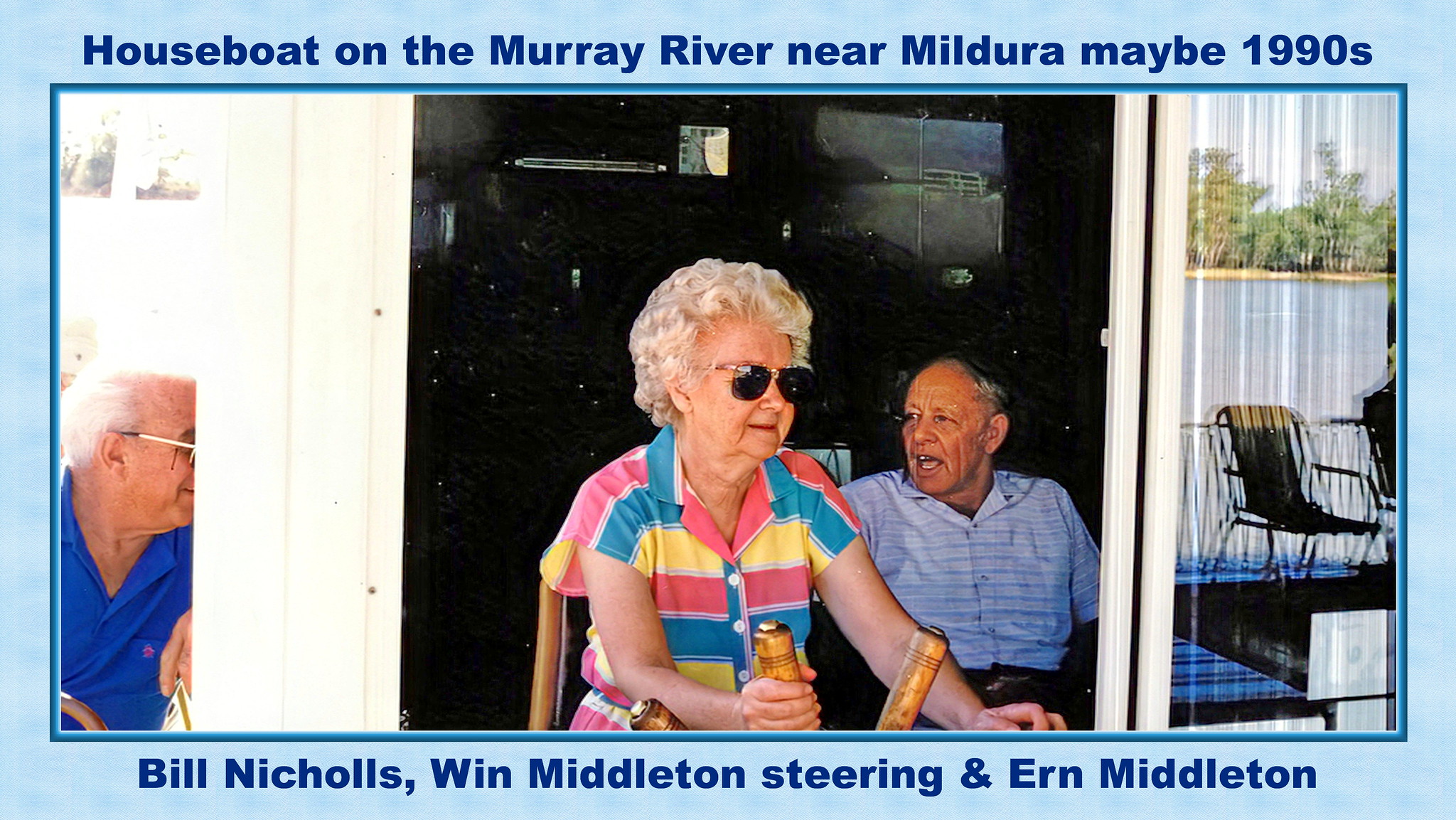The photograph appears to be taken on a houseboat named along the Murray River near Mildura, possibly in the 1990s. It features a woman with white hair and sunglasses, wearing a colorful shirt consisting of blue, pink, and yellow hues. She is standing up, holding a wooden steering wheel that looks like it belongs on a boat. Positioned behind her is a man in a blue t-shirt with a large liver spot on his cheek, seemingly engaged in conversation with another man. To the left, partially obscured by a vertical white rectangle, is an elderly man with white hair and glasses. The backdrop resembles a house's porch but is, in fact, part of the houseboat. Additionally, the image includes a black background with a picture resembling a waterfall in the top right corner. The far right side shows a beach chair and some trees. At the top of the photograph, it’s labeled “Houseboat on the Murray River near Mildura, maybe 1990s,” with the names "Bill Nichols," "Wynne Middleton Steering," and "Ern Middleton" listed below. 

This detailed caption captures the essence of the photograph, highlighting the key elements and contextualizing the setting and subjects involved.